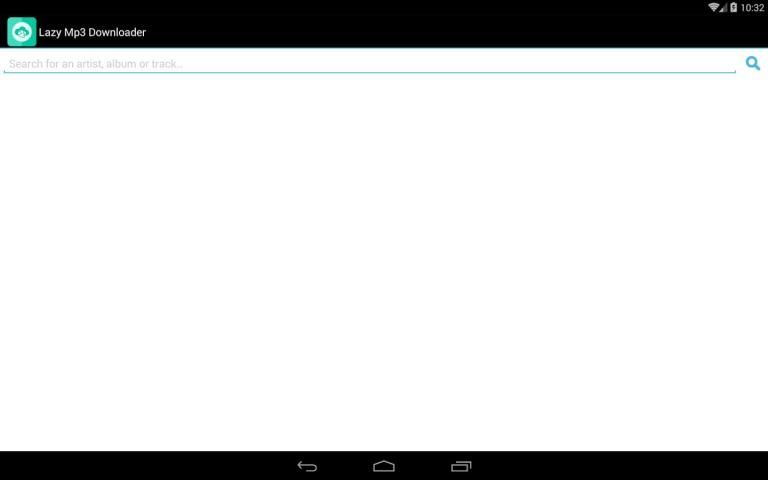This image is a screenshot from a website interface. At the top, a black banner spans the width of the page. Positioned in the top-left corner of the banner, the text "Lazy MP3 Downloader" is prominently displayed in white. On the top-right corner, there are three icons in white: a Wi-Fi signal indicator, a battery symbol, and the time displayed as "10:32".

Beneath the black banner lies a broad expanse of white space, dominated centrally by a search bar prompting the user to "search for an artist, album, or track". At the far right end of this search bar, a blue magnifying glass icon indicates the search functionality.

Further down, more white space extends towards the bottom of the image. Near the very bottom, another black horizontal bar stretches across the screen. This bar includes, in sequential order from left to right, an arrow pointing to the left, a house icon symbolizing the home page, and a rectangle that may signify additional options or a menu.

Additionally, a small green square is placed in the top-left corner of the white space, containing a white circle within which there is an icon resembling a tree.

There are no photographic elements, animals, or automobiles present in this image.